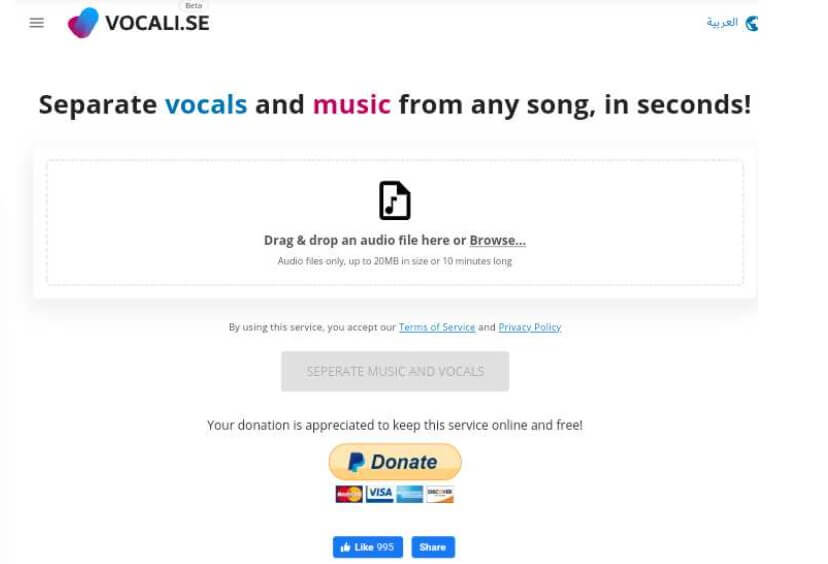This image is a detailed screenshot from a website with a clean white background. The top header is also white, featuring the company's name on the left, spelled "V-O-C-A-L-I dot S-E" in bold, black, capital letters. To the left of the company name, there is a logo consisting of two overlapping circles—one blue and one purple—forming a shape reminiscent of the letter "V".

Beneath the header, the main headline reads "Separate Vocals and Music from Any Song in Seconds." The word "Vocals" is in the same blue as the logo, and "Music" is in the same purple, while the rest of the text is in black.

In the center of the screenshot, there is an outlined square with a black musical note icon. Below this, the text says "Drag and drop an audio file here or browse," prompting users to upload a file.

Further down, a message informs users that "by using the service you accept our terms of service and privacy policy," with "terms of service" and "privacy policy" as blue hyperlinks. Additionally, a gray text note states, "Your donation is appreciated to keep the service online and free," next to a gold "Donate" button featuring the PayPal logo—a blue letter "P" with a light blue shadow.